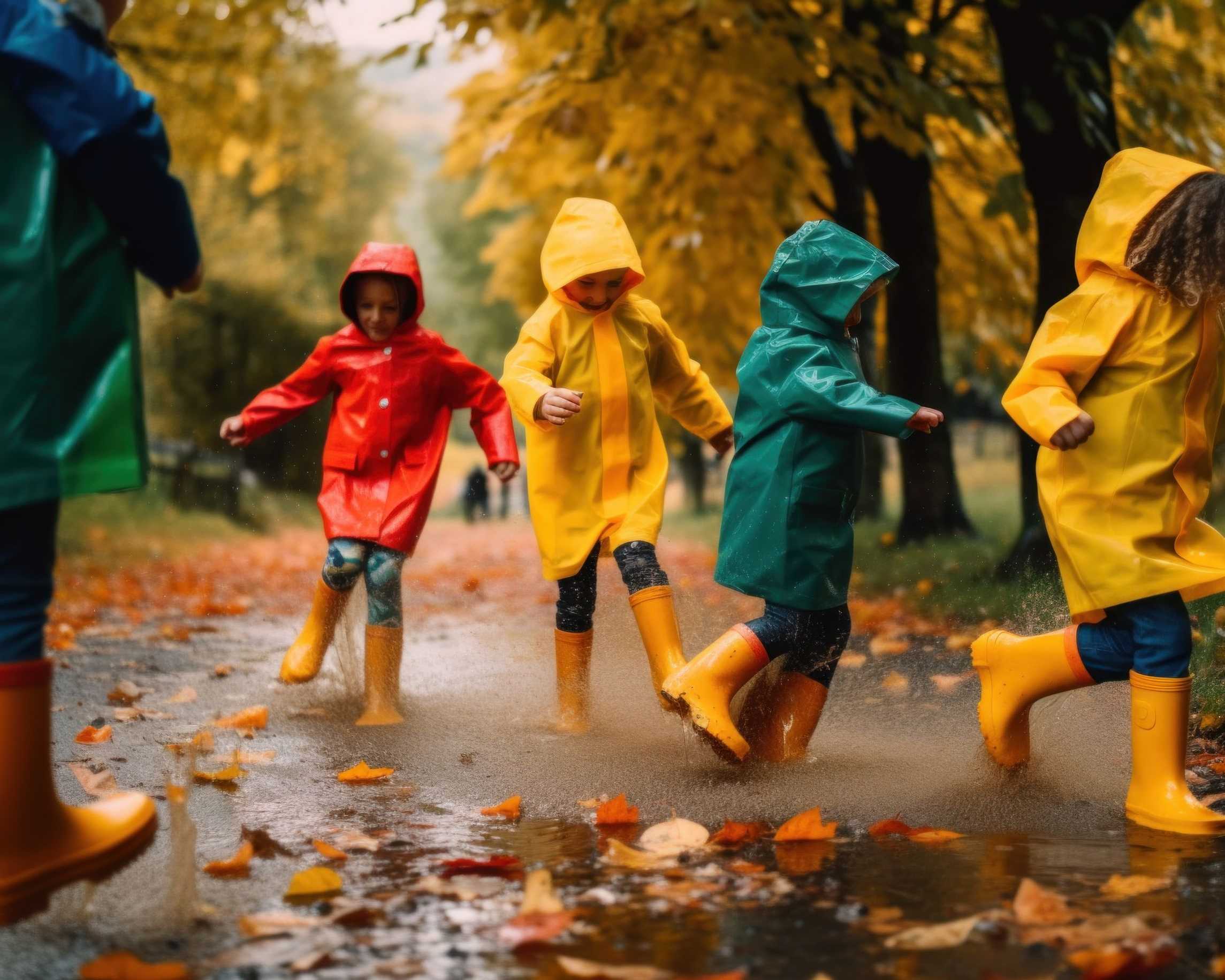On a typical rainy autumn afternoon in a park, four children clad in colorful raincoats and yellow rain boots joyfully splash and stomp in a large puddle. The ground is scattered with fallen leaves, enhancing the fall ambiance. The child on the far left wears a red raincoat, while the one next to her dons a yellow raincoat. Continuing left, there's a child in a greenish-teal raincoat, followed by another in a yellow raincoat. Off to the side, a figure in a green raincoat with yellow boots—possibly another child or an adult due to perspective—joins in the fun. In the background, blurred figures of other park-goers fade into the bokeh. The scene is vibrant with splashes of water from raindrops and playful energy under the autumnal trees shedding their leaves.